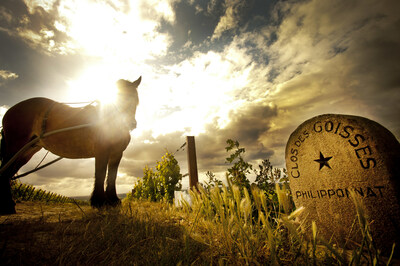This outdoor photograph, taken from ground level, captures a pastoral scene lit by intense sunlight behind a four-legged animal, possibly a horse or miniature pony, which casts a long shadow to the left. The horse, positioned on the left side of the image, is heavily silhouetted by the bright sun that peeks over its neck, creating a halo effect. The sky is speckled with numerous white clouds against a backdrop of dark blue. On the right side of the image stands an old-style, curved-top tombstone inscribed with the text "Clos des Goises Philipponat" and a star symbol. The immediate area around the tombstone is dotted with green grass, hay, or lighter grass, and there's a hint of a wooden post with wires, possibly part of grapevines in a vineyard setting. The scene is serene yet dramatic, with the bright sunlight creating stark contrasts and deep shadows throughout the photograph.